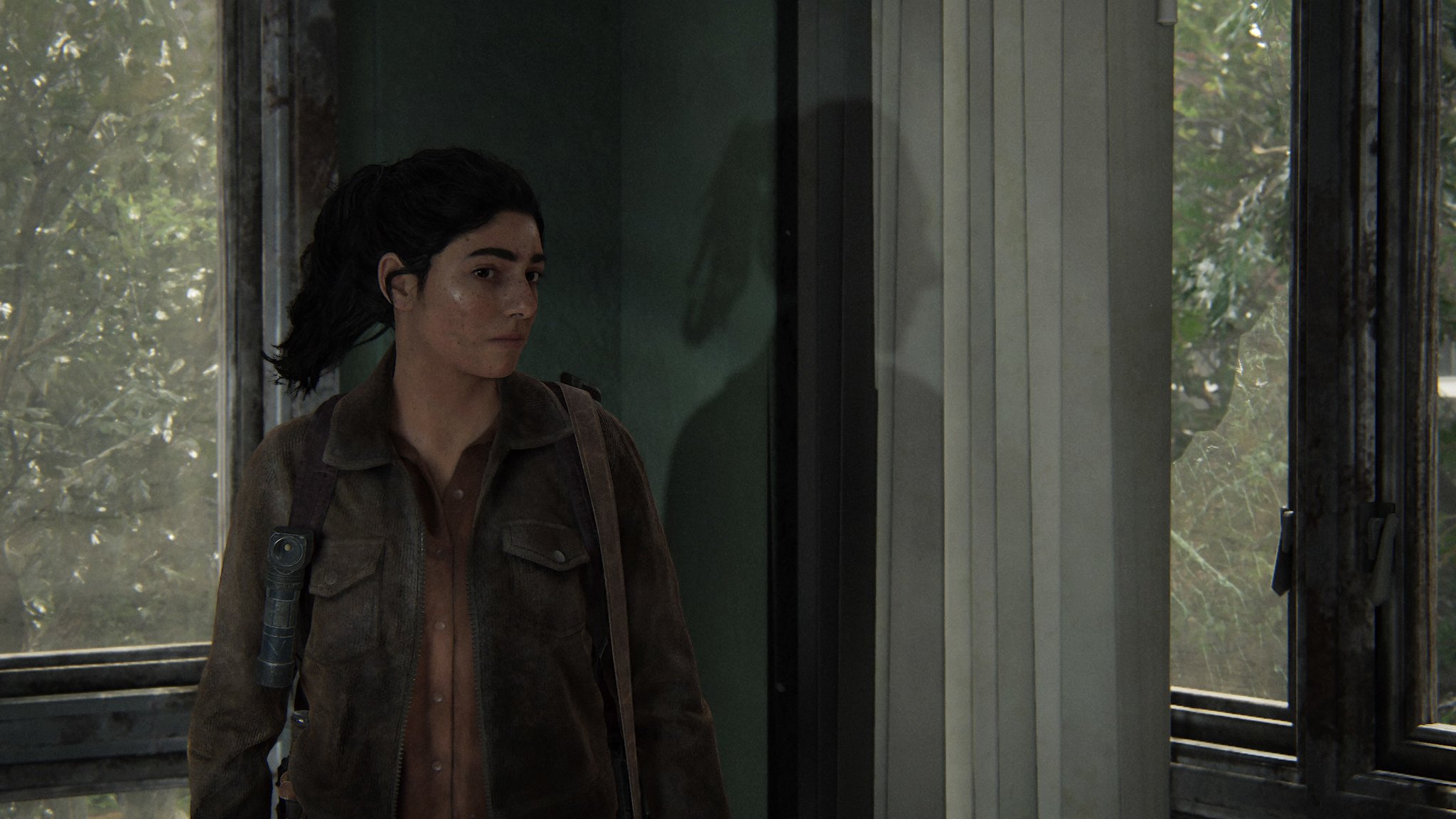This image appears to be computer-generated, depicting a scene either from a video game or a highly realistic animation. The focal point is a woman with fair skin, dark eyebrows, and dark hair tied into a ponytail that ends just above her shoulder. Her expression is neutral yet slightly downturned, suggesting a hint of defiance or caution. She is clad in a dark olive jacket with two front pockets over a brown button-up shirt, the top button left undone. Strapped around her shoulders is a backpack, potentially containing survival gear indicative of a post-apocalyptic or zombie-themed setting. 

She stands in a corner, flanked by two windows. One of these windows, partially obscured by vertical white blinds, offers a glimpse of an outdoor scene suggesting dusk or early evening, with two trees faintly silhouetted. The wall behind her is predominantly green, contrasting with another white or faintly depicted pane, possibly a painting. Her stance and setting evoke a sense of alertness, as if she is either hiding or preparing for some imminent threat. Elements such as a suspected firearm strapped under her arm and additional gear on her backpack further enhance this tense, survivalist atmosphere.